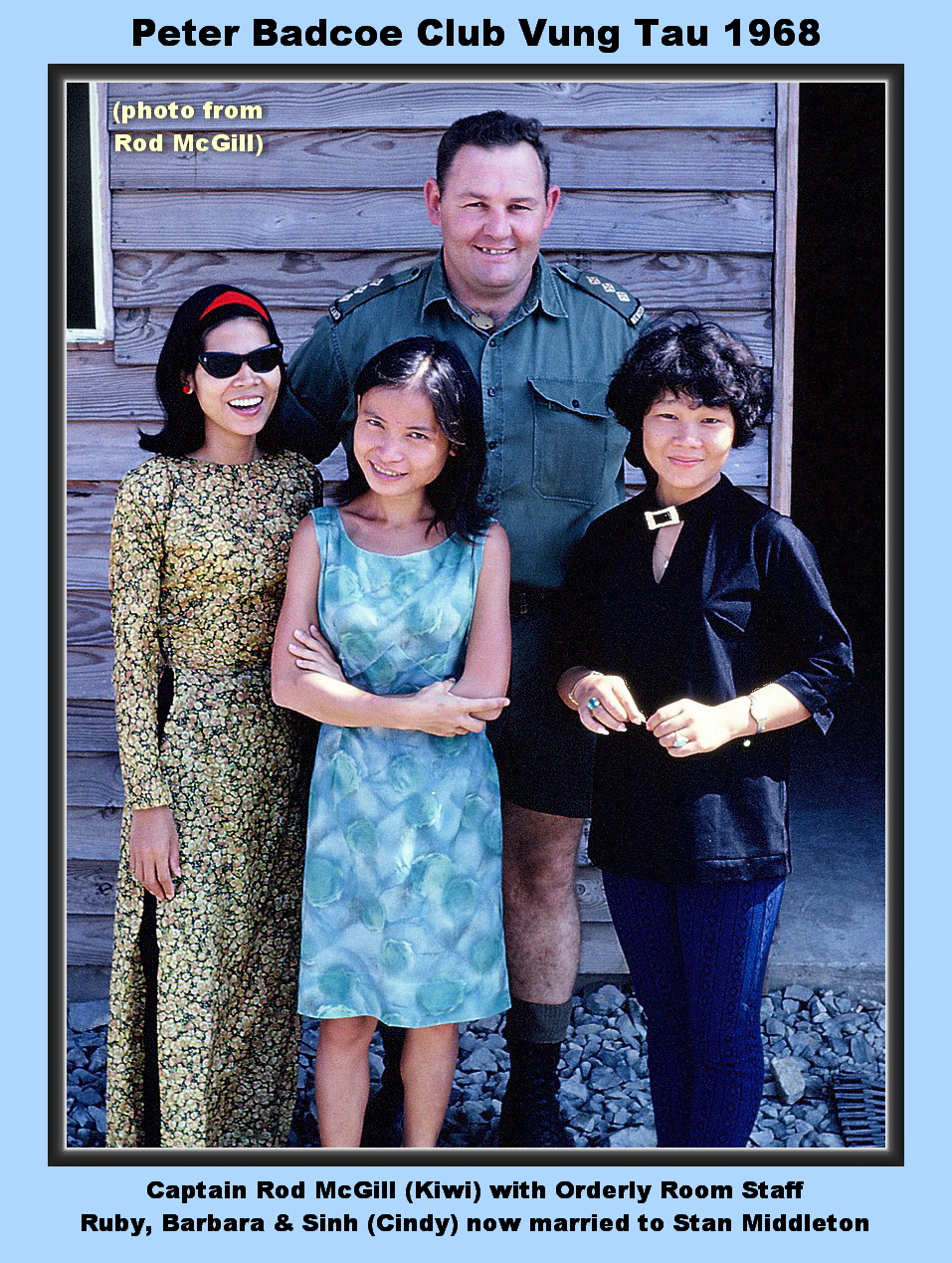This vertically aligned, full-color faded photograph, set against a light blue border with a dark gray inner frame, captures an outdoor scene during the day in 1968 at Club Vung Tau. The background features wooden siding, slats, and possibly the end or entryway of a building, with the far-left edge showing part of a window. The ground is strewn with small rocks.

In the image are four individuals: a tall white gentleman, identified as Captain Rod McGill (Kiwi), wearing a green military uniform top, black shorts, and boots, smiling at the camera. Accompanying him are three Asian women, likely Vietnamese. The woman on the left, Ruby, sports a gold-pattern dress, a red headband, shoulder-length black hair, and black sunglasses, smiling broadly. In the center, a young girl named Barbara is dressed in a blue and white floral dress with her arms crossed and head tilted down slightly, yet smiling. The woman on the right, Sin (Cindy), now married to Stan Middleton, wears a black shirt and blue jeans, with short black hair and a smile.

Above the picture, black text reads: "Peter Badko, Club Vung Tau, 1968." Below, the caption details "Captain Rod McGill (Kiwi) with orderly room staff, Ruby, Barbara, and Sin (Cindy), now married to Stan Middleton."